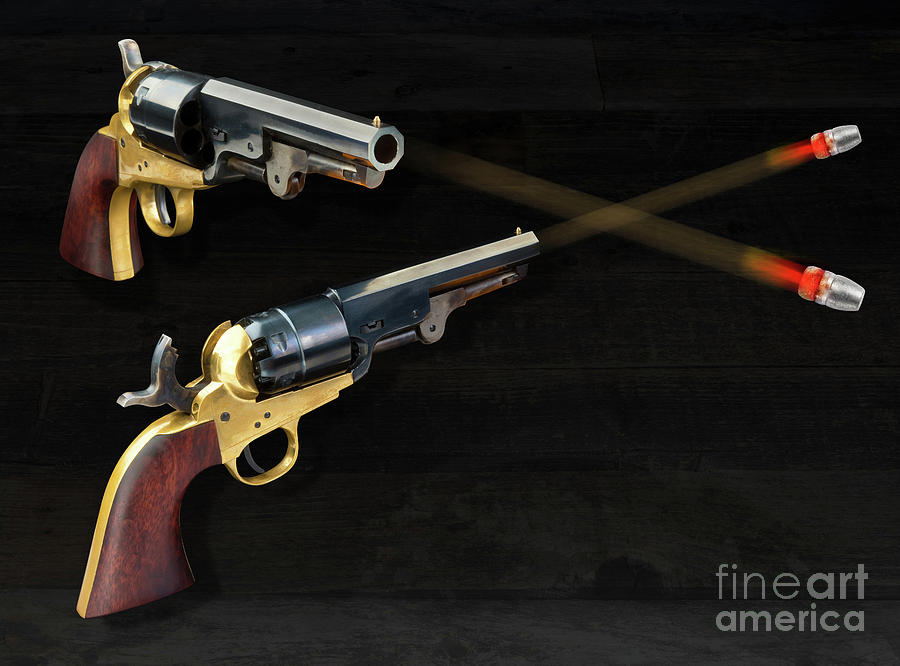The image depicts a dynamic scene of two vintage revolvers firing bullets diagonally so that their paths cross without colliding. Each gun has a distinct red-brown wooden handle with a golden accent and features a rusted iron or brass hammer, while the barrel and bullet chamber are black. The bullets, with silver tips and red bases emitting red jet effects, leave light orange streaks marking their trajectories across a black background that resembles a charcoal wood plank and bears visible brush strokes. The artistic rendition, noted for its colorful detailing, has a watermark in the lower right that reads "fineartamerica" in lowercase, vividly emphasizing both the historical elegance of the revolvers and the dramatic action of the firing sequence.